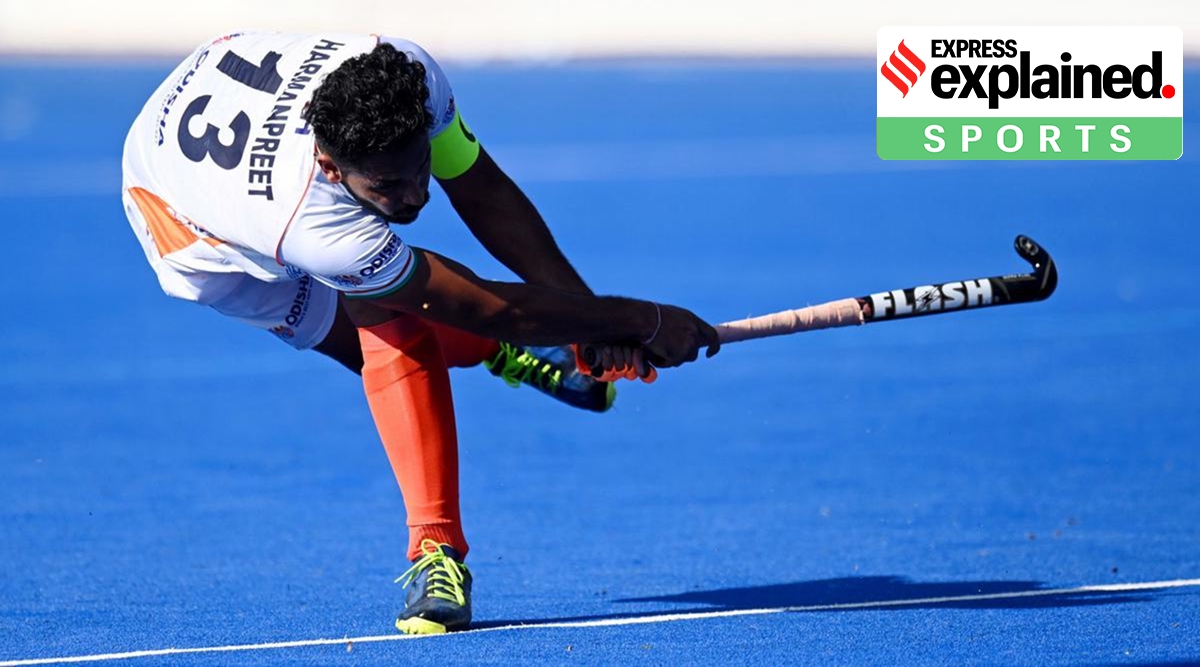The image depicts a dark-complexioned male field hockey player, probably around 30 years old, actively engaged in a game. He is captured mid-swing on one leg, his right leg extended straight behind while his bent left leg touches the bright blue artificial turf. He grips a short, curved hockey stick labeled "Flash" with both hands, and his momentum hints at the possibility of a fall. The player wears a white jersey and matching white shorts, with the name "Harmanpreet" and the number 13 emblazoned on the back. His outfit is completed with orange socks, shin guards, and blue shoes with neon yellow laces. Adding to the professional look, the image includes a post-production label at the top right reading "Express Explained Sports," indicating it is likely from a sports periodical. The vibrant blue field has clearly marked white lines, highlighting the dynamic nature of the sport being played.